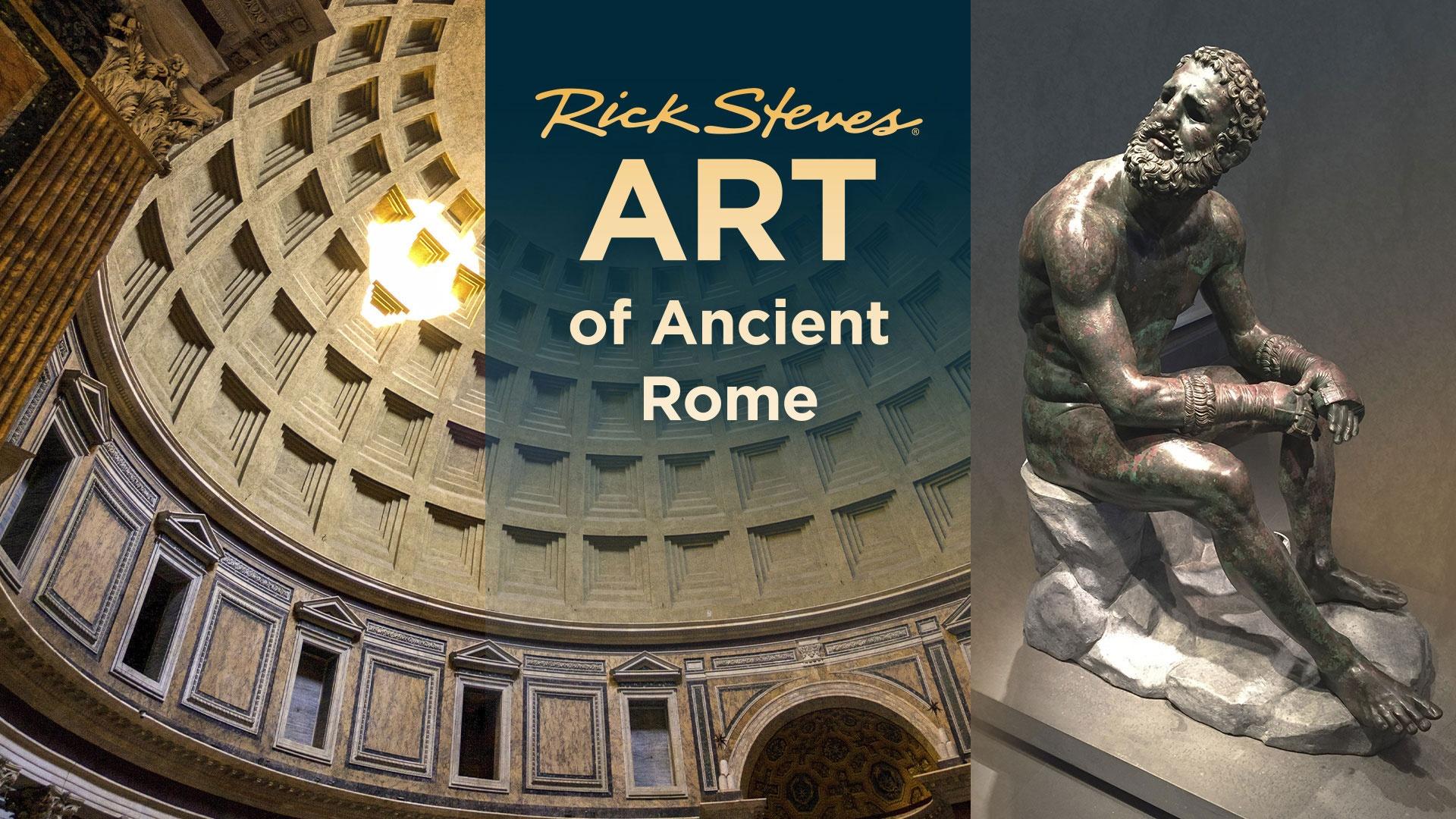This image is an advertisement or flyer for an art exhibit titled "Rick Steves Art of Ancient Rome," prominently displayed in white text at the center on a green background. The backdrop features the interior of a historical, dome-like structure reminiscent of a museum, constructed from marble and adorned with embedded squares for texture. The dome is grandiose with light filtering through the top, creating a luminous effect. Flanking the central text are brown and gold pillars or posts. To the right, the flyer showcases a bronze sculpture of a muscular nude man seated on a stone, characterized by a full beard and extremely curly hair. The figure is depicted in a contemplative pose, gazing upward, distinct from the well-known Thinker statue. On the upper left side, there seems to be an additional sculpture, possibly of two figures, enhancing the artistic ambiance of the flyer.